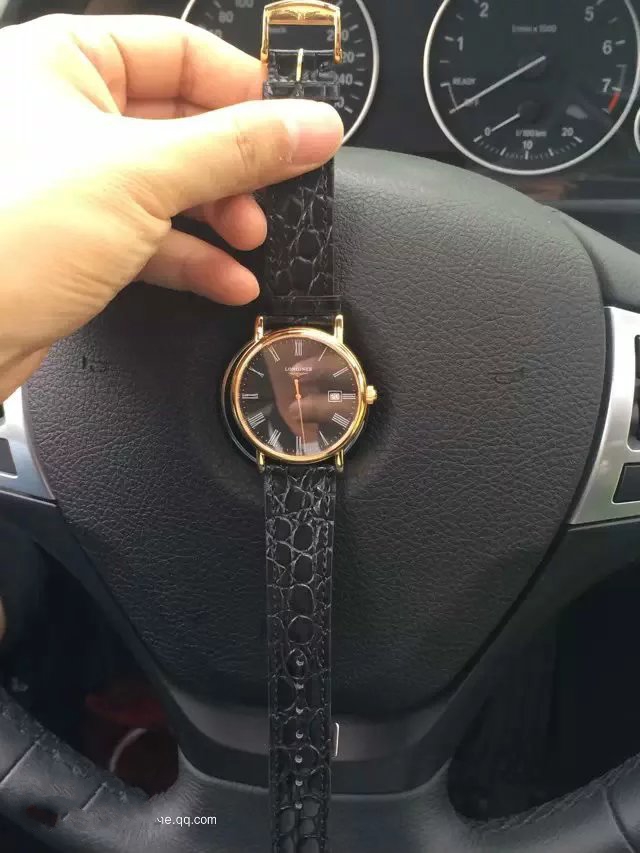The image captures a surreal first-person POV of an individual holding a wristwatch over the center of a car's steering wheel, with their left hand. The watch, perfectly aligned with the horn button at the center of the wheel, has a black leather strap textured to look like crocodile or snake skin. The clasp and the pendant, including a knob on the right side, are all gold. The circular gold frame encases a black face showcasing white Roman numerals, a logo at the top middle, and an additional small digit indicator. The watch hands, also gold, point to around 5:29. In the reflection of the watch’s glass face, you can observe two fingers wrapped around a phone, suggesting that the photo is taken by the individual's right hand. The black steering wheel and part of the car's dashboard, including the speedometer at zero, are visible in the background, indicating the car is stationary. Additional details include the text "QEW.QQ.com" on the bottom middle-left of the watch face and hints of a rev counter on the dash.